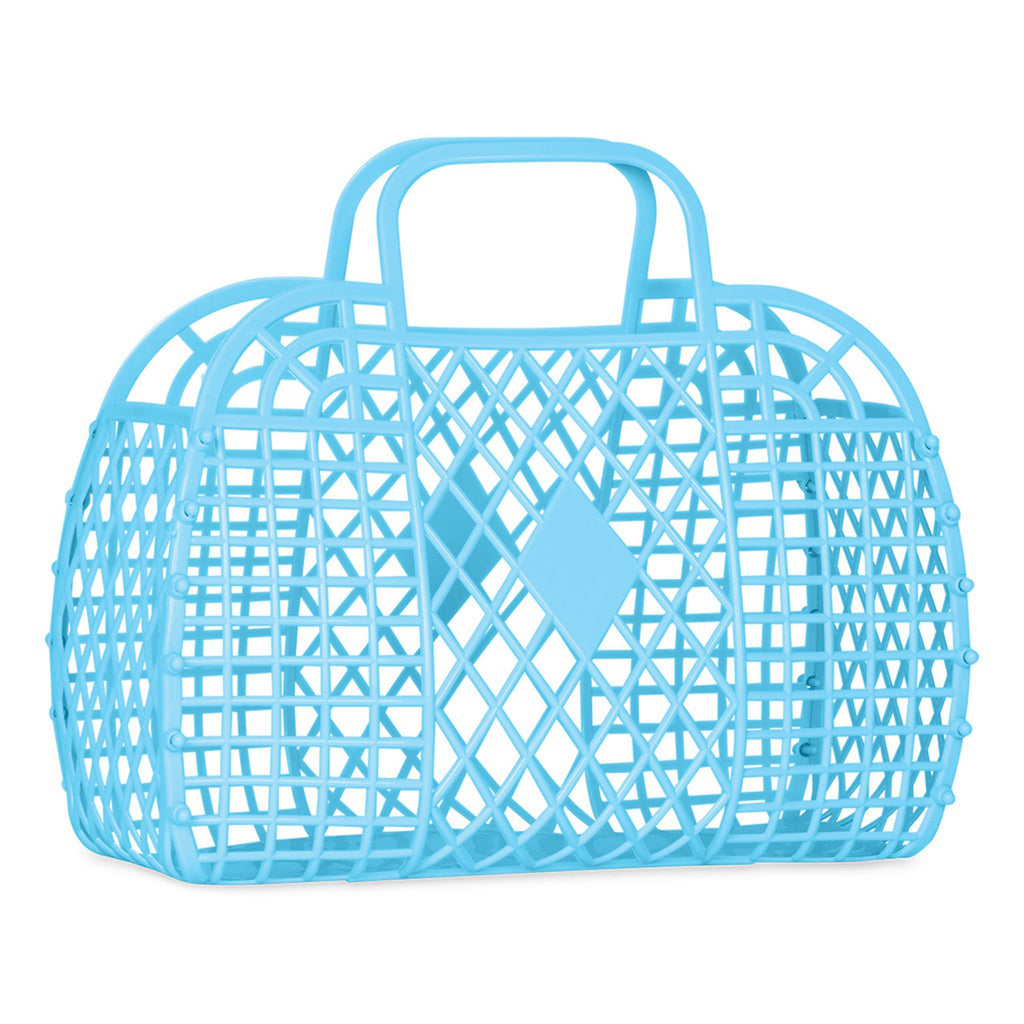This illustration depicts a soft, lightweight blue jelly purse, appearing almost like an outline with transparent sections that create a crisscross, diamond-patterned mesh design. The cotton candy-colored purse is empty and positioned to showcase its long side, making it perfect for an advertisement or website display. Its two thin plastic handles and see-through structure suggest it's versatile for carrying lightweight items, potentially suitable for beach essentials like sunscreen. The decorative rhombus patterns filled in blue add a unique touch, giving the purse a delicate and airy aesthetic. The overall design hints at an origin from China, emphasizing simplicity and functionality.